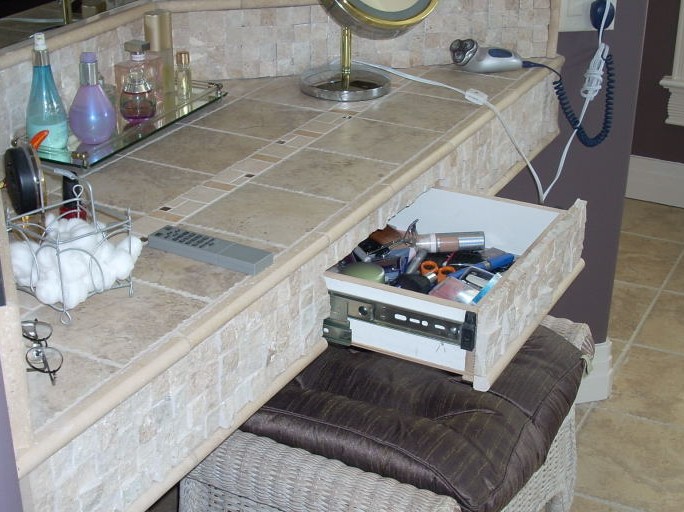This image features a cozy and uniquely shaped makeup vanity, nestled into a niche with a trapezoidal layout. The vanity is adorned with a large mirror and has an open drawer, revealing an array of makeup products inside. Below the drawer, there's a cushioned stool in a rich purple hue. The surrounding walls share this purple theme, creating a harmonious and inviting space. Additionally, a handheld mirror sits nearby, ready for use.